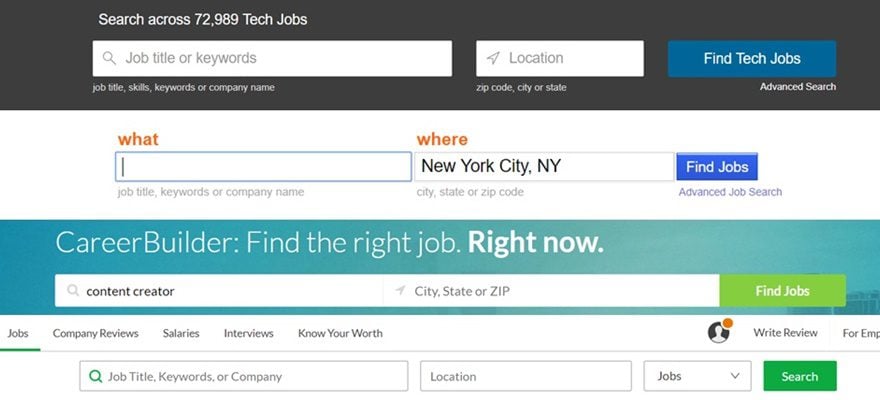The image features a prominently displayed search interface on the CareerBuilder website. At the top, there is a rectangular, dark gray banner with white text that reads, "Search across 72,989 tech jobs." Below this banner, there is a white search bar section. On the left side of this section is a small gray magnifying glass icon followed by the text "Job title or keywords." To the right, there's another box labeled "Location" with a small navigation arrow icon, and next to it is a blue button that says "Find Tech Jobs." Below the search bar, “Advanced search” is written in white text.

Under the "Location" box, the text "zip code, city, or state" is shown in lowercase letters without an Oxford comma. Similarly, on the left side under the "Job title" text, "job title, skills, keywords, or a company name" is spelled out, also missing an Oxford comma.

Below this search bar section, there's a white banner with the word "What" written on it. It features a static search bar with a permanently displayed cursor, leading to some uncertainty about whether it is interactive. Inside the search bar, the text reads "job title, keywords, or company name." To the right, the search location is set to "New York City, New York," in a search box labeled "city, state, or zip code."

Further down, a bluish-green banner has white text at the top saying "CareerBuilder:" utilizing a capital "C" and "B." The banner text reads, "Find the right job. Right now." Below this text, there's another search bar. "Content creator" is entered in the left side of the search bar with a magnifying glass icon next to it. To the right, the location box has the same small navigation arrow and reads "city, state, or zip," with a green "Find Jobs" button.

At the bottom of the search interface, there is a navigation menu. The "Jobs" tab is selected and highlighted with a green underline. Next to it are tabs for "Company Reviews," "Salaries," "Interviews," "Know Your Worth," and others including a person icon and an abbreviated section labeled "EMP," likely for "Employers."

The bottommost section contains another search bar with a green magnifying glass icon and prompts for "job title, keywords, or company." The location box stands to the right of this with a "Jobs" dropdown arrow, followed by a green button on the far right.